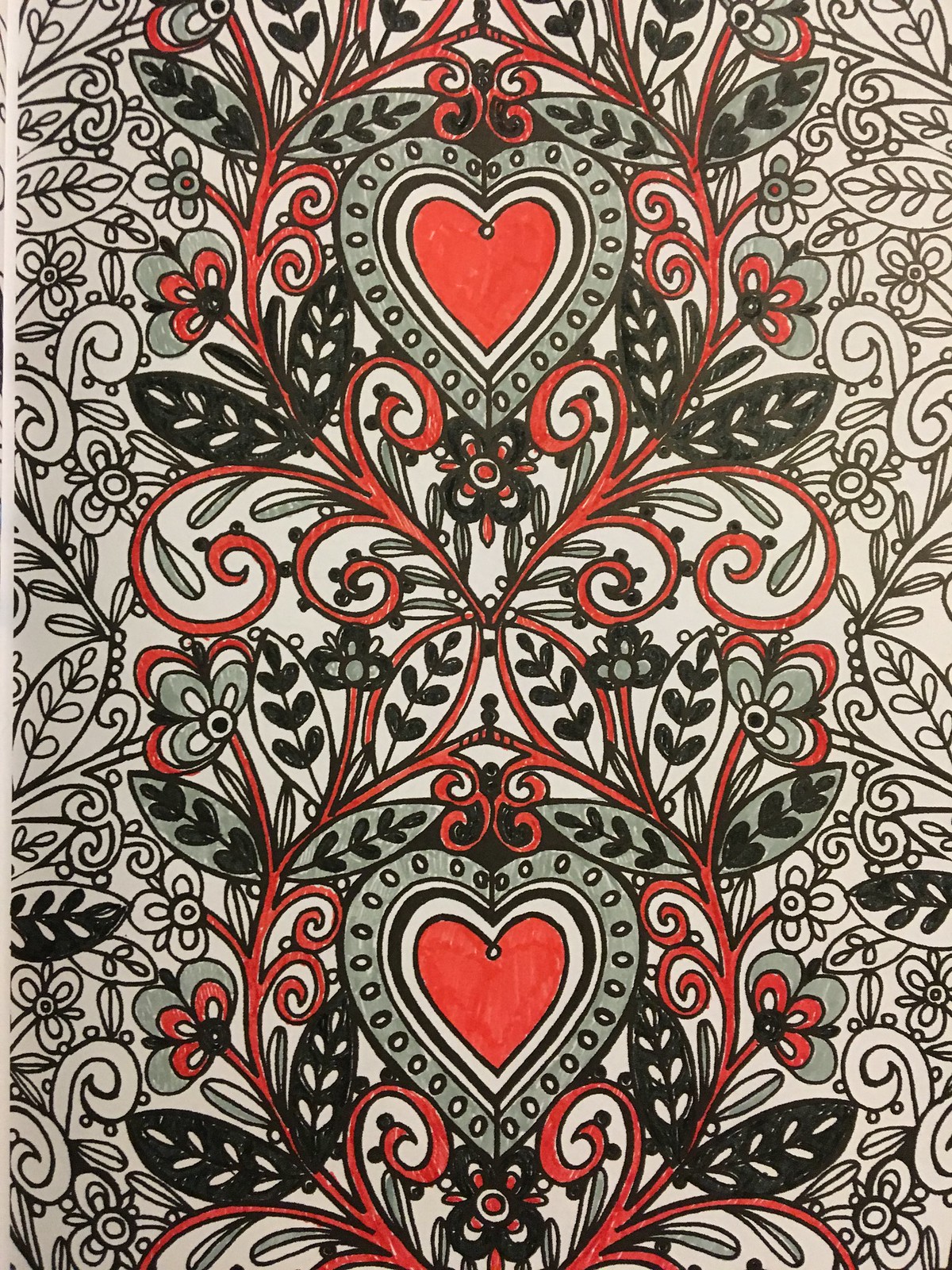A vibrant and colorful image, likely sourced from a coloring book, showcases a variety of elements meticulously colored in with marker. At the heart of the image are several hearts, featuring a rich red center and encircled by a pristine white border. Surrounding these hearts is a gray background adorned with evenly spaced white dots. Beneath this central motif, there are stylized black leaves marked with intricate white patterns. The image also includes elegant fleur-de-lis curlicues, adding a touch of sophistication to the composition. Although the central part of the picture has been fully and vividly colored, many flowers and other elements around the periphery remain untouched, retaining their original black and white outline. The artist's attention has clearly been concentrated on the central section, leaving ample space for further creativity.